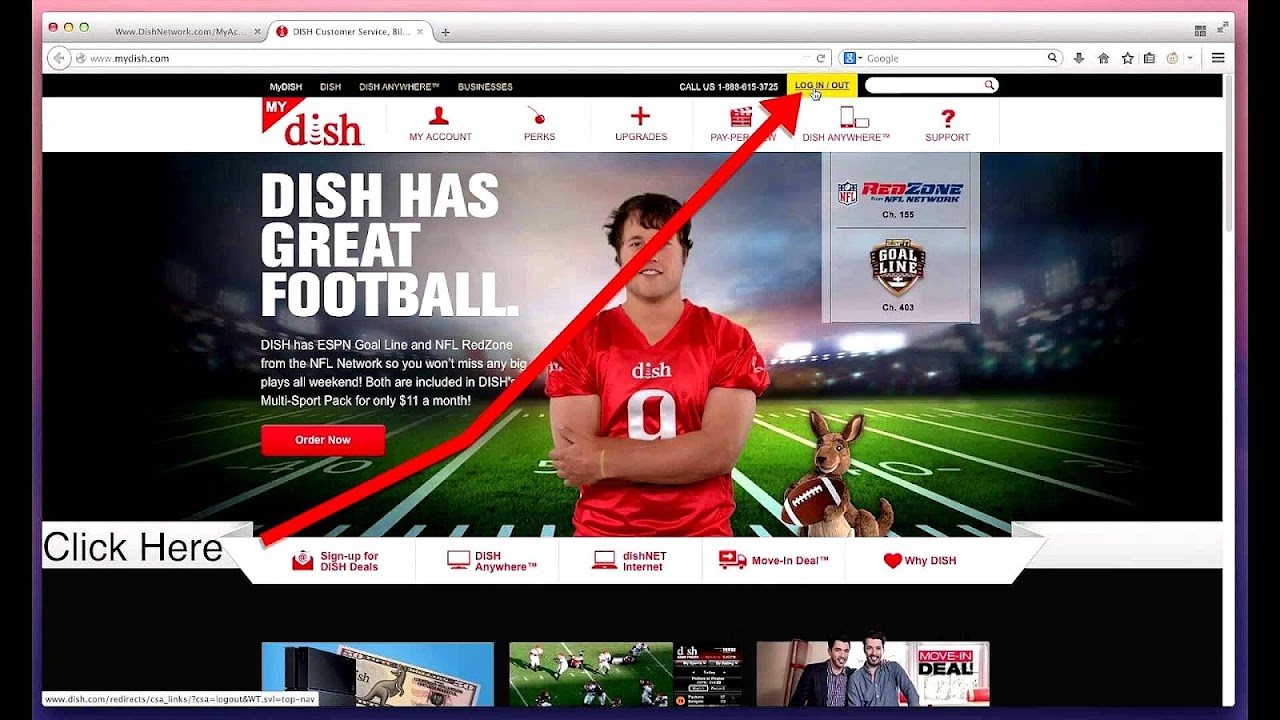In the center of the image, the focal point is a man wearing a bright red football jersey with the word "Dish" emblazoned across the middle, followed by a number. He has short, dark hair, and his arms are confidently crossed in front of him. To his side is a small toy kangaroo holding a football. A long, red arrow originates from a "click here" prompt in the lower left corner and extends across the man's face, pointing towards a yellow box at the top right that encourages you to click it.

Adjacent to the man's image, the text reads, "Dish has great football. Dish has ESPN, Goal Line, and NFL Red Zone from the NFL Network. So you don't want to miss any big games." Below this text is a prominent red square containing the words "Order Now." Above this informational area is the Dish logo in red, alongside options for "My Account," and "Upgrades," marked with a plus sign, located to the right. On the far right of the image, the word "Support" is accompanied by a question mark above it.

At the bottom of the image, there are additional options to sign up for "Dish Deals," "Dish Anywhere," "Move In Deal," and "Why Dish," the latter represented by a heart symbol.